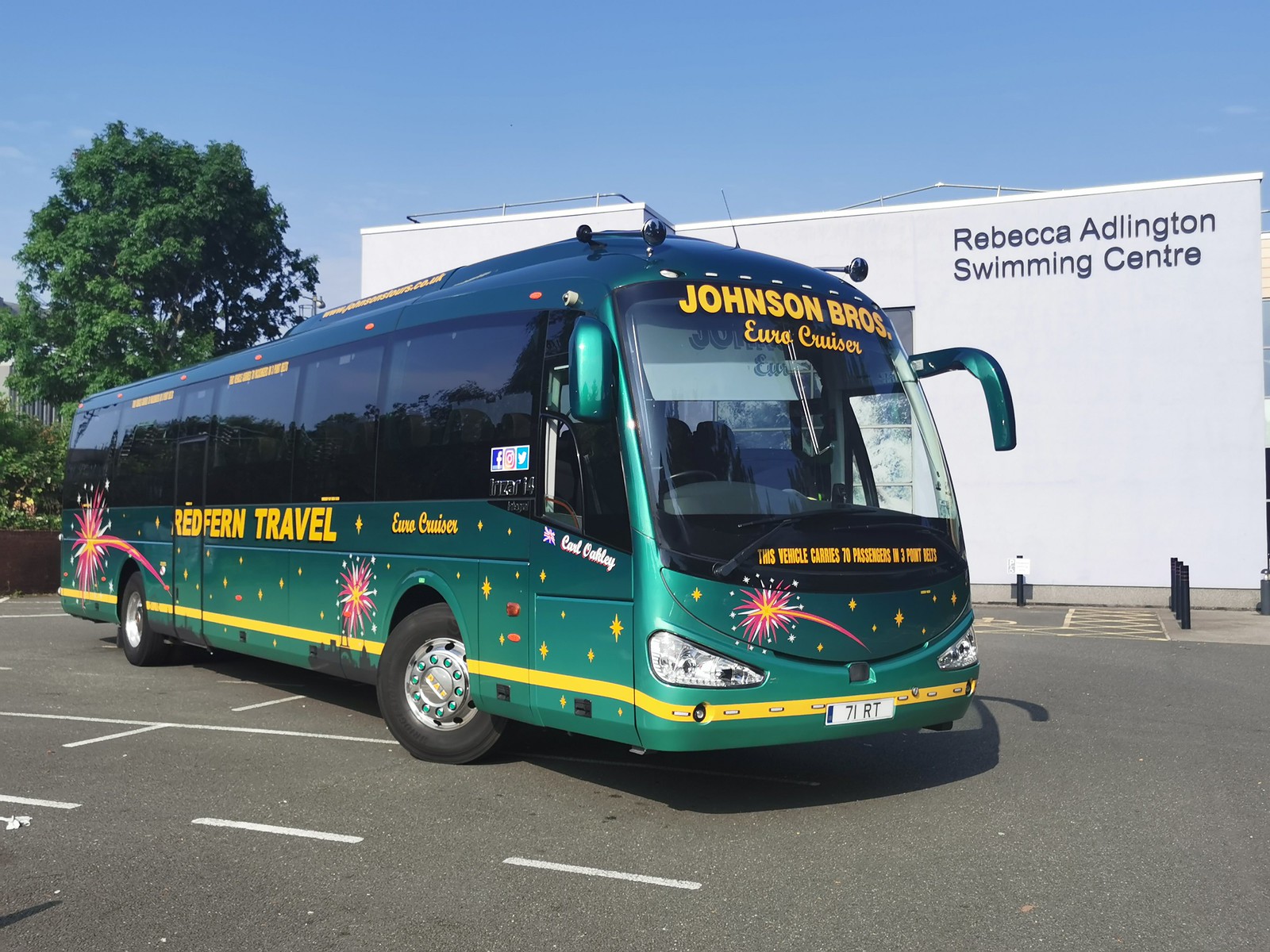In the image, a large, predominantly green bus gradually transitions from a darker shade at the top to a lighter green at the bottom. The bus, which belongs to the travel agency Red Fern Travel, features vibrant illustrations of fireworks and stars along its sides. Prominent text on the side identifies it as a "Redfern Travel Euro Cruiser," and the front displays "Johnson Bros Euro Cruiser" alongside the bus license plate 71RT. The windows are dark-tinted and adorned with labels indicating social media icons for Facebook, Instagram, and Twitter, suggesting modern connectivity.

The bus is empty and parked in a largely vacant parking lot, situated near the Rebecca Adlington Swimming Center. There is a large tree with lush green leaves on the left side of the image, adding to the scenic surroundings. The detailed artwork and text on the bus, along with the substantial size, highlight its capacity to carry up to 70 passengers, likely indicating its use for large group travel, potentially including swimmers, given its location next to the swimming center.